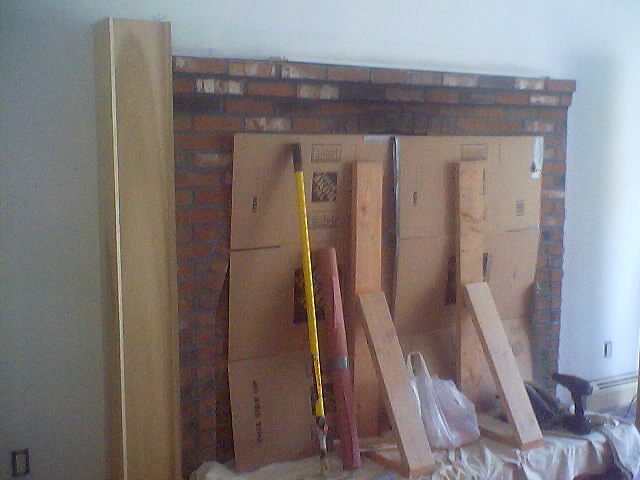The image is a low-resolution color photograph showing a partially refurbished indoor brick fireplace set against a pixelated and discolored white wall. The grainy image reveals greenish and pinkish tones due to poor camera quality. Central to the scene is a red brick fireplace with unevenly colored bricks, including patches of white, dark brown, and black. The fireplace is covered by two vertically positioned sheets of cardboard, propped up by light brown vertical planks and tan-brown diagonal planks at 45-degree angles against the floor. In the foreground, a dust sheet covers the base of the fireplace, with various tools scattered around. To the left of the right vertical plank, a yellow painting pole is visible, while on the right side, atop the dust sheet, sits the black silhouette of a power tool, likely a drill. Additionally, there are cylindrical objects wrapped in red with silver accents, and a small white bag is noticeable. Electrical outlets without cover plates are visible on both the left and right sides of the scene, the left one near the corner, enhancing the sense of ongoing renovation.